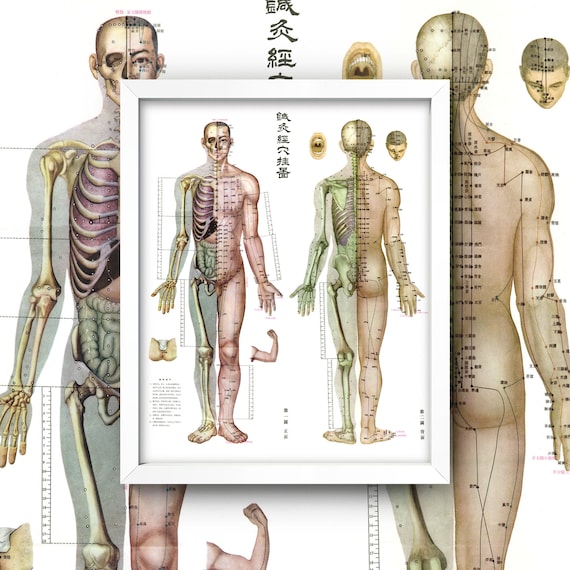The image is a highly detailed illustration of human anatomy, specifically focusing on a male figure. The central composition features a framed inset image that replicates the larger, background depiction. On the left side of the figure, the interior structures are visible, revealing the bones, organs, and muscles. The face shows flesh and hair, while the rest of the body exposes the ribcage protecting the pink-colored lungs, the olive green stomach, and part of the leg with visible bones. In contrast, the right side of the figure presents the skin fully intact, extending from the head to the feet, with the individual facing away from the viewer. Intricate details punctuate the image, including various measurements and annotations in a language different from English, likely Chinese, that highlight different regions and elements of the body. The juxtaposition and framing emphasize the anatomical contrasts between the skeletal, muscular, and integumentary systems.